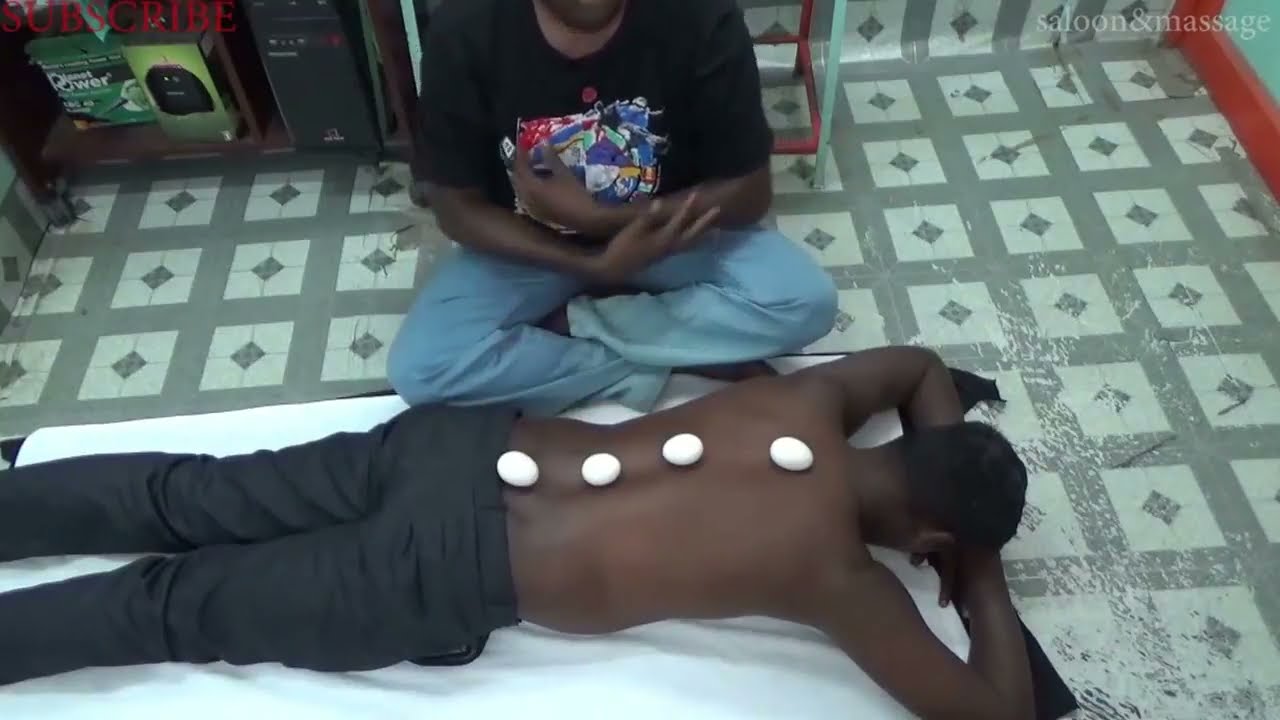The image depicts a scene where a shirtless man with dark brown skin, possibly of Indian descent, is lying face down on a small white mattress. His head is resting on his hands, and he has black or dark blue pants on. There are four white, oval-shaped stones placed along his spine, from the upper back to the lower back, suggesting he is undergoing a treatment. The room has a tiled floor with a light green and dark green square pattern.

Directly above him in the image, there's another man with dark brown skin, also likely Indian. This man is sitting cross-legged on the ground, wearing a black T-shirt with an obscured logo and light blue jeans. The background features a green-tiled wall and a shelving unit to the left, which contains various indistinguishable items. At the top left of the image, the word "subscribe" appears in small red font, and at the top right, the words "saloon and massage" are written in light white font.